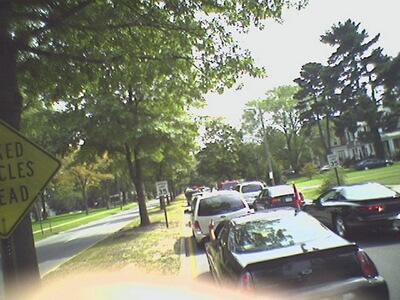This photograph captures a suburban street on a sunny day, teeming with traffic. In the center, numerous small compact sedans are either moving or closely parked, except for a single white SUV situated amongst them. These vehicles are following closely, maintaining a distance of about five to ten feet from each other, giving the appearance of a traffic jam. The street is flanked by tall, bright green trees that tower almost three times the height of a prominent white house visible in the top right corner. Road signs on both sides indicate a speed limit of 35 miles per hour. Separating the traffic is a green median filled with trees that also line the opposite two-lane road running in the opposing direction. The sky above appears cloudy, but the day remains bright, illuminating the greenery and road ahead.